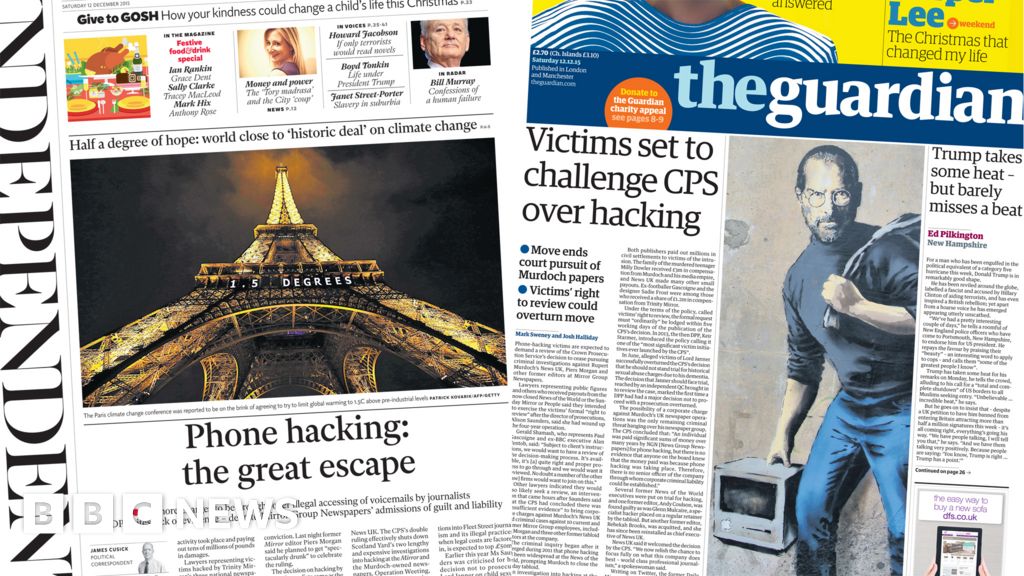This image displays a collage consisting of two newspaper front pages. On the left is the newspaper titled "The Independent," with the name printed vertically along the left side in large black capital letters. The focal point of this cover is a photograph of the Eiffel Tower, set against a dark gray background. Beneath the image, there is a prominent headline in black text that reads: "Phone Hacking: The Great Escape."

On the right side of the collage is the front page of "The Guardian." This cover features a yellow border at the top, with the newspaper’s title, "The Guardian," written below it on a blue background. Directly under the title, on the left side of the page, is a headline in black text on a white background stating: "Victims Set to Challenge CPS Over Hacking." Adjacent to this headline, on the right side, is a photograph of a man resembling Steve Jobs, dressed in glasses, a black turtleneck, and denim. 

The composition of the collage emphasizes the juxtaposition of the two newspaper covers, both addressing topics related to phone hacking.